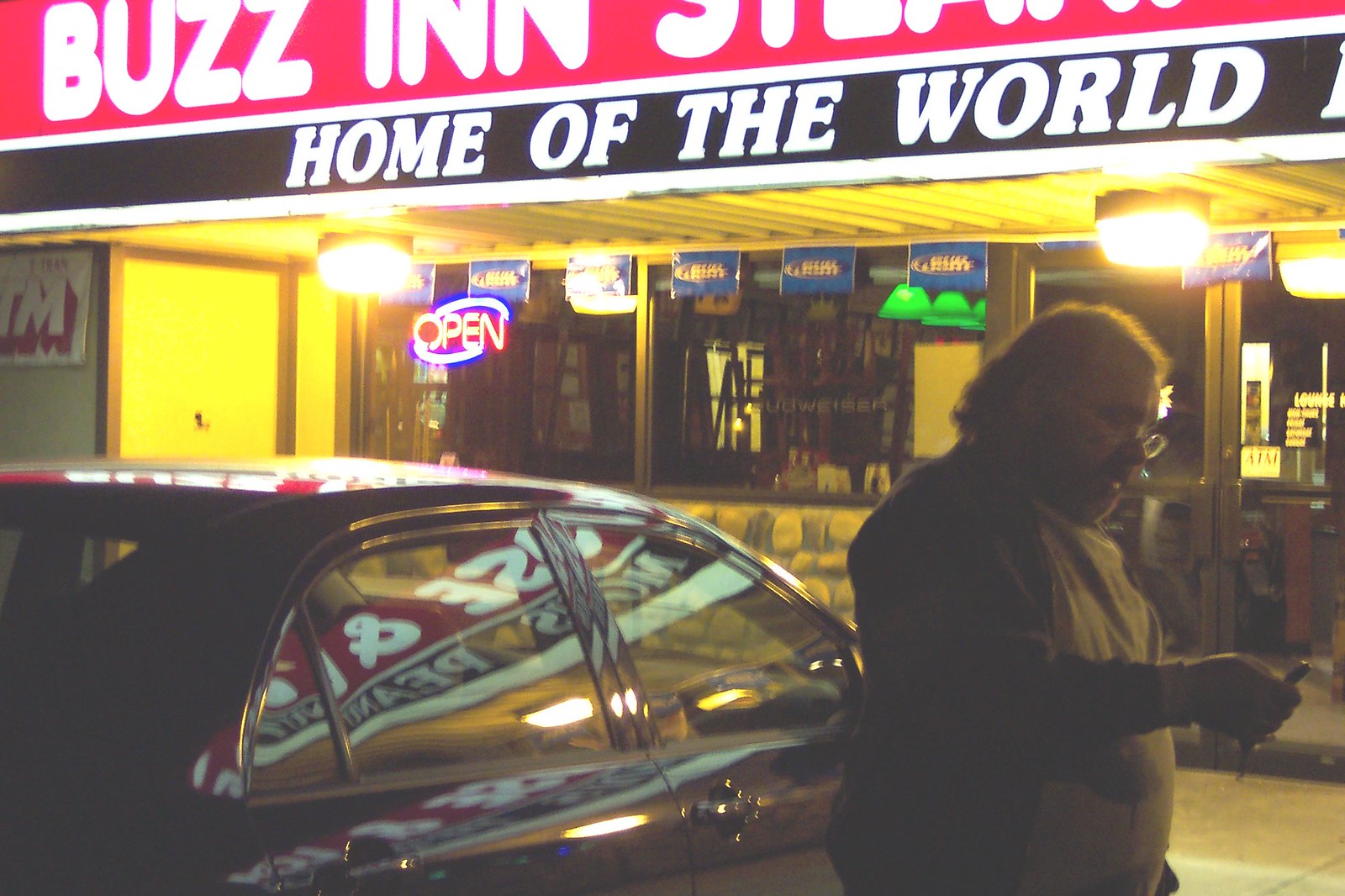The photograph features a night-time scene outside a brightly-lit liquor store with a prominent, partially cropped red sign displaying "Buzz Inn" in white letters against a red background. Below this, another sign reads "Home of the World" in white letters against a black background. The store has a neon "OPEN" sign in red and purple, glowing in a window to the left of the main entrance, which is flanked by two bright lights on the ceiling casting an orange glow. The entrance consists of double glass doors with a black frame, adorned with various Budweiser signs.

In the foreground, a heavier set, middle-aged man with glasses is standing beside a shiny black car, holding his key fob in his right hand, appearing to lock the vehicle. His side profile shows him looking downward, partially illuminated by the store's bright lights. He wears a long-sleeve shirt that appears grayish under the store's illumination, and his hair is short in the front and long in the back. The reflective surface of the car and the store’s illuminated signs and windows create a vivid contrast with the dark surroundings.